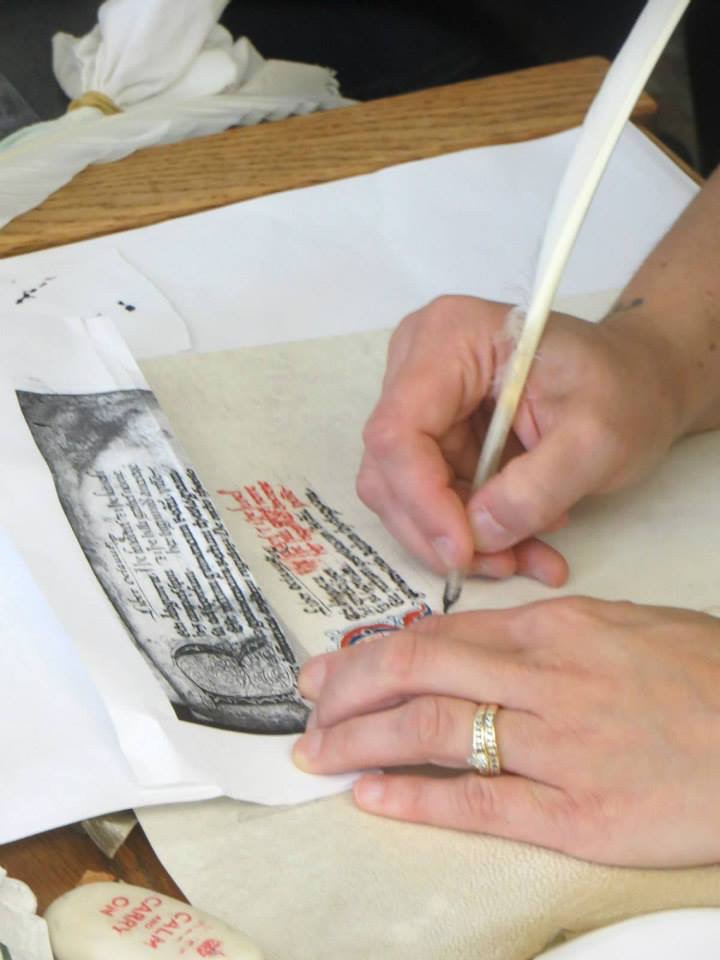In the photograph, a person is seated at a light brown desk, engaged in the meticulous task of transcribing calligraphy. They are using a white feather quill pen in their right hand, tracing medieval-style cursive on a piece of light cream, semi-transparent parchment. This page is being copied from a black and white reference sheet above it. Their left hand, adorned with a silver wedding ring and a larger ring set with diamonds, rests on the desk. The desk is lined with a white cloth, which has ink stains from the quill. In the top left corner of the image, there's a bundle of white napkins wrapped in a rubber band. In the bottom left, a white, roundish container with red lettering sits, likely an eyeglass case that reads "keep calm and carry on." The background includes a white surface and possibly a black chair or object, adding depth to the scene.